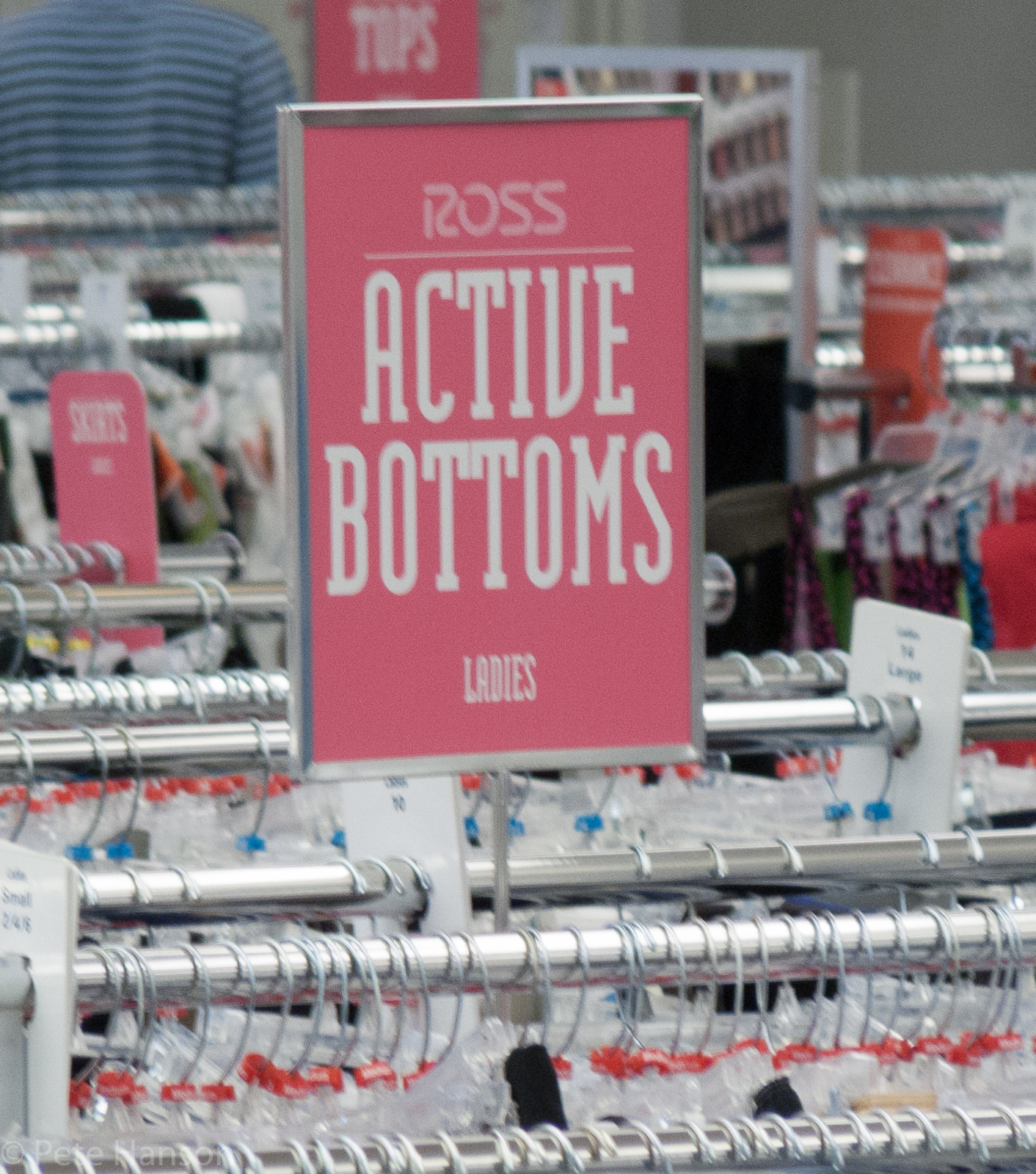This detailed image captures the interior of a retail store, specifically a Ross Dress for Less, as evidenced by the signage. Prominently displayed is a square sign framed in silver chrome. The sign itself features the Ross logo above the words "Active Bottoms" in red text, with a smaller inscription reading "Ladies." Beneath this, chrome racks filled with various garments can be seen. The hangers, adorned with red and blue plastic size markers, indicate the size range of the clothing. Additionally, white signs on the hangers specify that the clothing size is large, providing clear size information for shoppers.